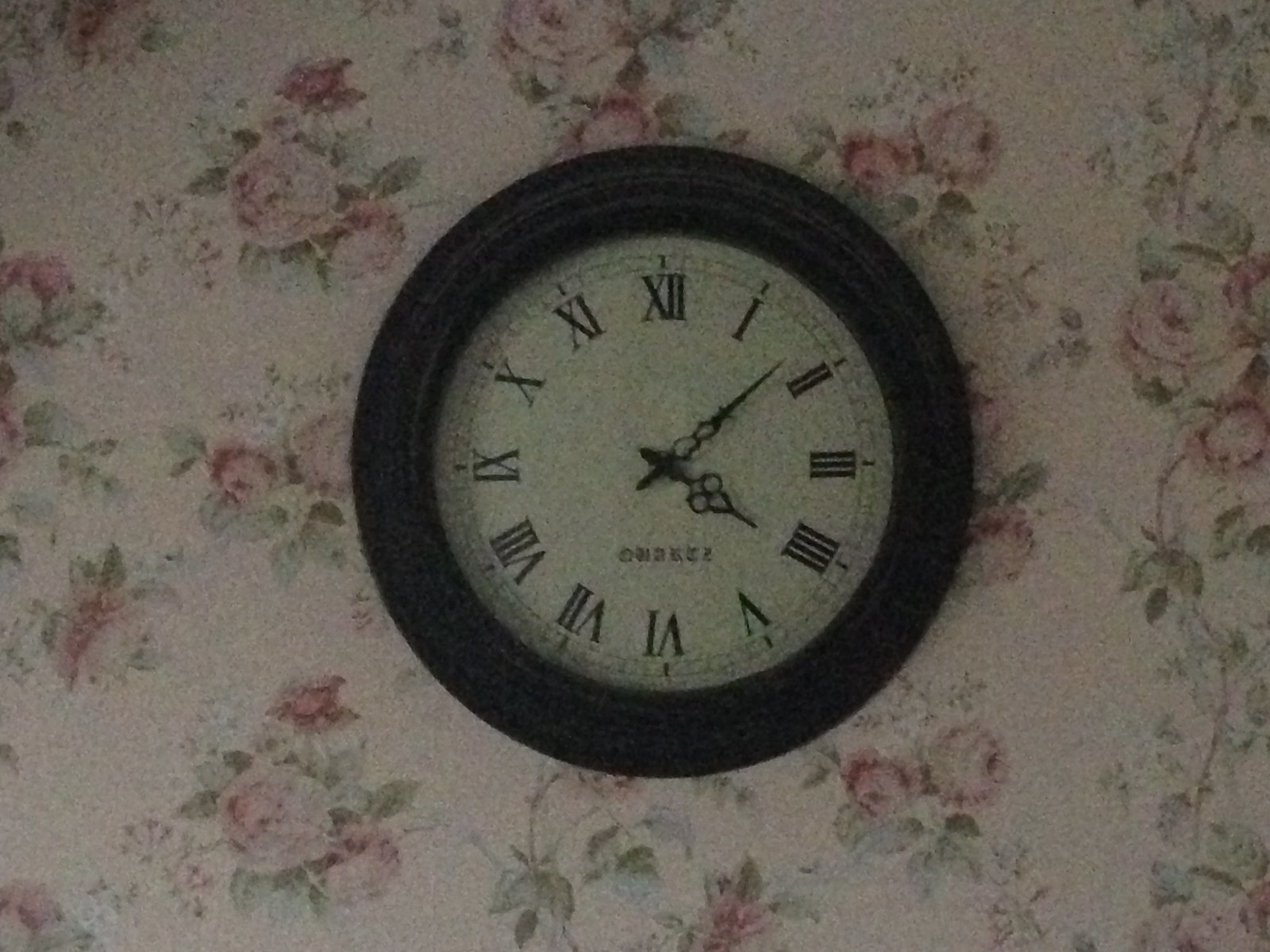This image captures a slightly blurred photograph of a round wall clock, encased in a black wooden frame. The clock is affixed to a wall adorned with pale pink wallpaper featuring an intricate pattern of pink roses, complemented by green stems and leaves. The clock's face is stark white, with striking black Roman numerals marking the hours. Both the minute and hour hands are crafted from black metal, featuring delicate, ornamental designs. Beneath the center point of the clock, there is some indecipherable writing, adding a touch of mystery. The clock stands alone on the wall, with no other items in proximity, giving it a solitary yet elegant presence in the grainy photograph.